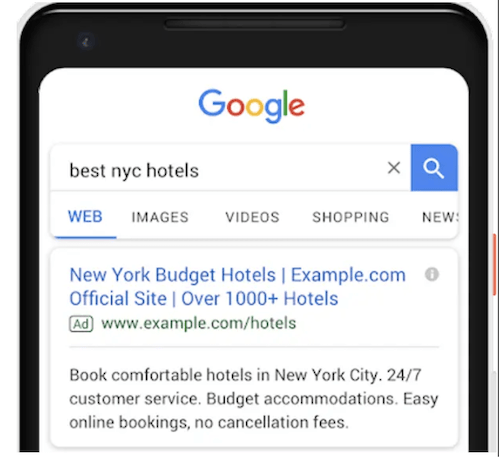The image captures a search result page on the Google website, displayed on a black device. The predominantly white background of the webpage features the Google logo prominently at the top, followed by a search box containing the query, "Best NYC Hotels." To the right of the search box is a magnifying glass icon, indicating the search function. Below the search box, several category tabs are visible: "Web," "Images," "Videos," "Shopping," and "News."

The first search result beneath these category tabs is highlighted as an advertisement. It presents the title "New York Budget Hotels" linked to the official site of "Example.com," which claims to have over 1,000 hotels available. The URL associated with this ad is www.example.com/hotels. Further details provided in the ad entice users to "Book Comfort Hotels in New York City," offering assurances such as 24/7 customer service, budget-friendly accommodations, easy online bookings, and no cancellation fees.